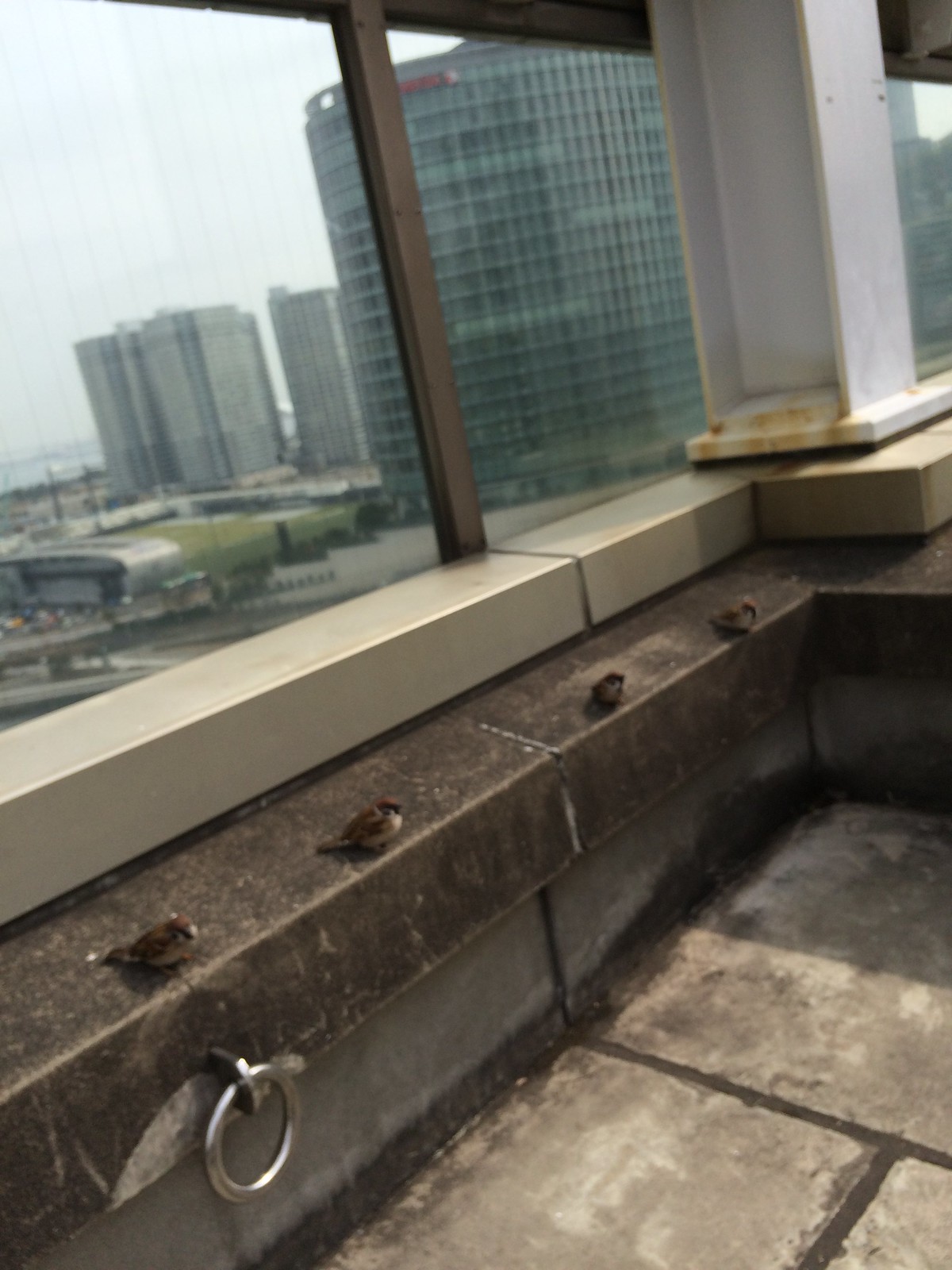The photograph showcases the rooftop corner of a tall building, offering a high vantage point over a bustling cityscape. The rooftop features a stone floor and is lined with a glass partition for safety. Prominently, a large white H beam is situated in the very corner, while a thick metal loop, likely for securing a chain, is visible in the foreground. The rooftop's edge, roughly 18 inches high and potentially suitable for sitting, is currently occupied by four small brown birds, probably wrens. The city below displays a mix of modern architecture, with several tall skyscrapers and office buildings, characterized by glass façades, one of which reflects its neighboring structures. The nearest building has a distinct greenish tint to its glass panels. Beyond the urban landscape, the sky is visible, and a river can be faintly discerned in the background, adding depth to the metropolitan view.